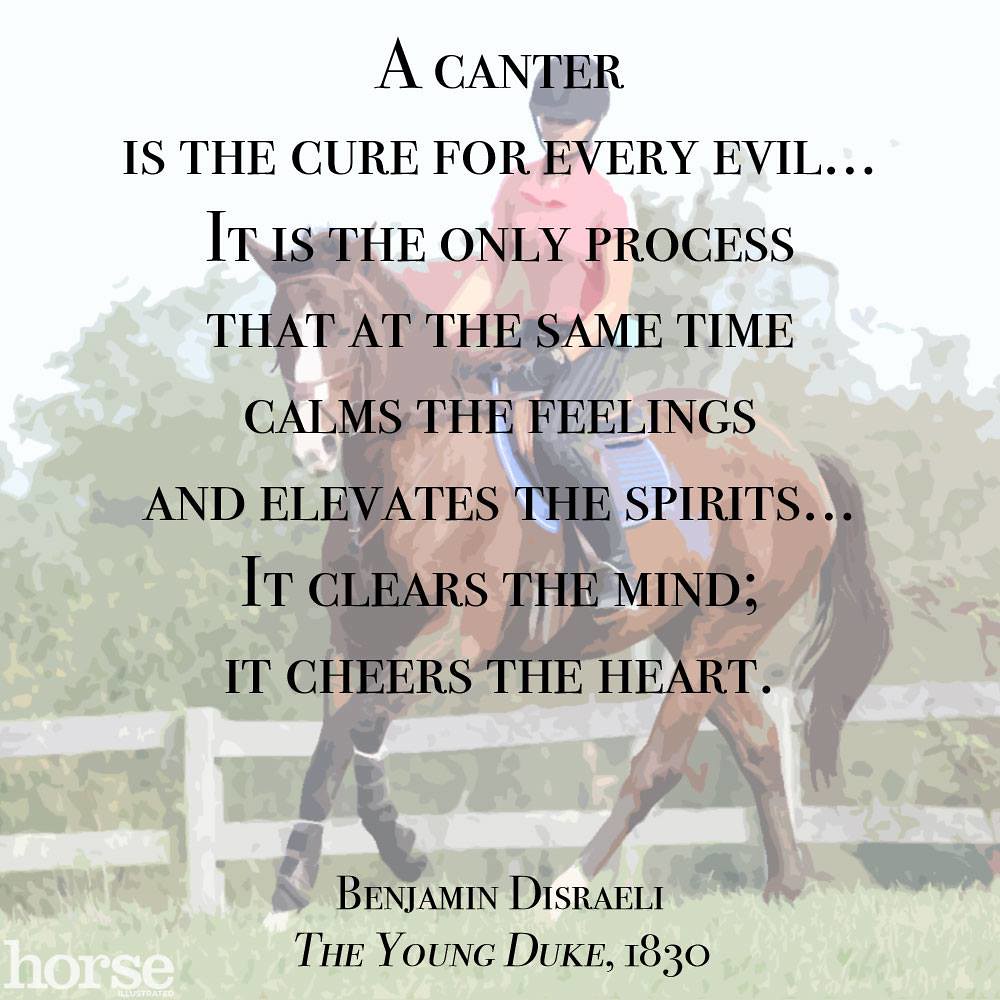The image features a detailed painting of a rider and her horse. In the foreground, a woman is riding a brown horse with a distinct white marking on its face. She is dressed in a pink polo shirt, black pants, black riding boots, and a black riding helmet. The horse is equipped with a brown saddle and a blue saddle blanket. The scene is set within a white picket-fenced area, and the background includes lush green surroundings and trees. Superimposed over this picturesque scene in black text are the words: "A canter is the cure for every evil. It is the only process that at the same time calms the feelings and elevates the spirits. It clears the mind. It cheers the heart. - Benjamin Disraeli, The Young Duke, 1830." Additionally, the bottom left corner of the image subtly includes the text "Horse Illustrated" in see-through font.